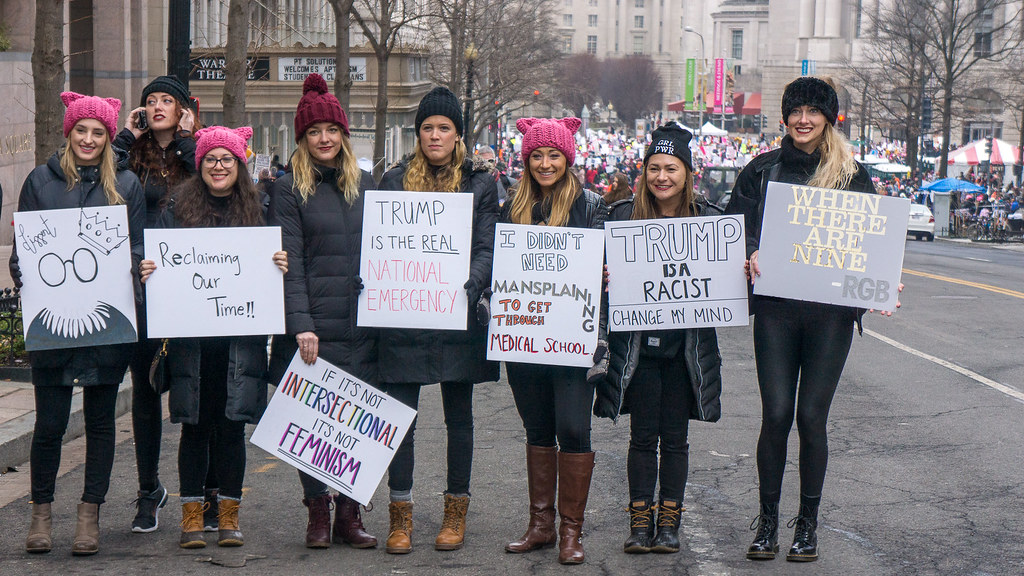In this outdoor, likely wintertime protest, a group of eight women is lined up, all dressed in warm clothing, including black jackets and various knit caps—three of which are pink with cat ears, while others are gray, black, or red. They stand on a cracked asphalt road that appears to have recently experienced rain or snow. Each woman is holding a sign with messages such as "Trump is a racist, change my mind," "I don't need mansplaining to get through medical school," "Trump is the real national emergency," "Reclaiming our time," and "If it's not intersectional, it's not feminism." One of the women is also on a cell phone. In the background, a cityscape with multiple buildings, including a theater, and a gathering of more people participating in some festivities are visible. The scene is adorned with trees, sidewalks, and canopies, enhancing the sense of a bustling protest in an urban environment.